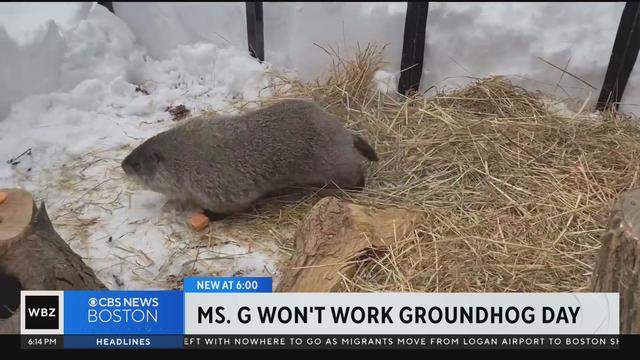The image is a color screenshot of a CBS News Boston broadcast, captured with the chyron reading "WBZ CBS News Boston" and "New at Six" on a blue background. Beneath this, a headline in black text on a white background states, "Mrs. G Won't Work Groundhog Day." The photograph features a small, brown groundhog in profile, facing left, within a cage or enclosure that contains some hay, a tree stump, and snow, indicative of a naturalistic setting. The cage appears to have black bars spaced wide enough for the groundhog to potentially escape. The scene suggests a typical Groundhog Day event, with the implication that Mrs. G, the groundhog, is refusing to participate in the day's traditional shadow-seeing activities.